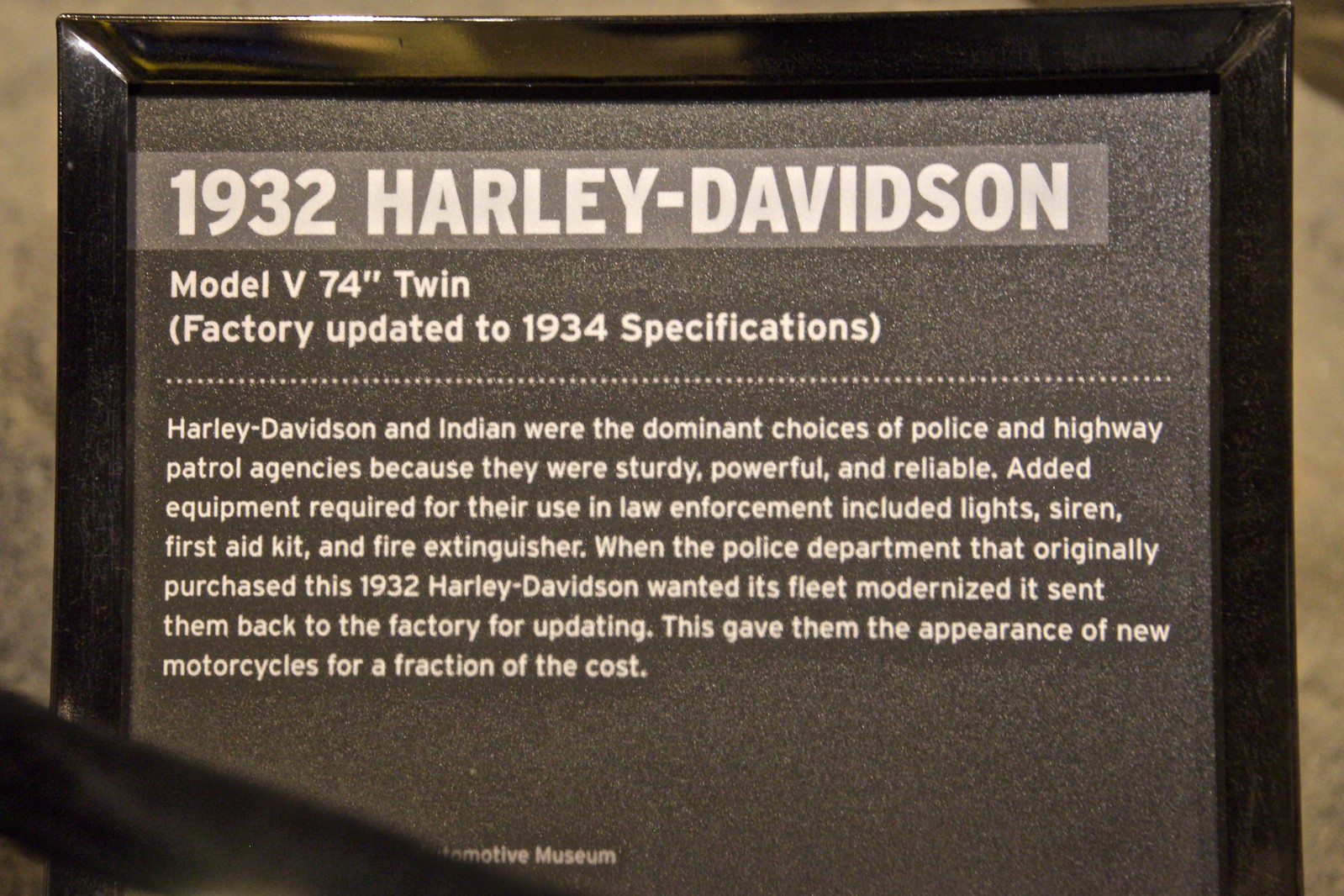The image depicts a framed plaque mounted on a wall, likely in a museum, with a black metal frame and a gray background. The top of the plaque prominently features the title "1932 Harley-Davidson" in bold white font, followed by a smaller, bold text that reads "Model V-74 Twin, factory updated to 1934 specifications." Beneath this is a detailed paragraph explaining that Harley-Davidson and Indian motorcycles were the favored choices for police and highway patrol agencies due to their sturdiness, power, and reliability. The plaque notes that additional equipment necessary for law enforcement use included lights, sirens, a first aid kit, and a fire extinguisher. It further explains that the police department, aiming to modernize its fleet, returned its 1932 Harley-Davidson motorcycles to the factory for updates, which provided the appearance of new motorcycles at a fraction of the cost. The plaque itself emits a notable glow, adding to its prominence.